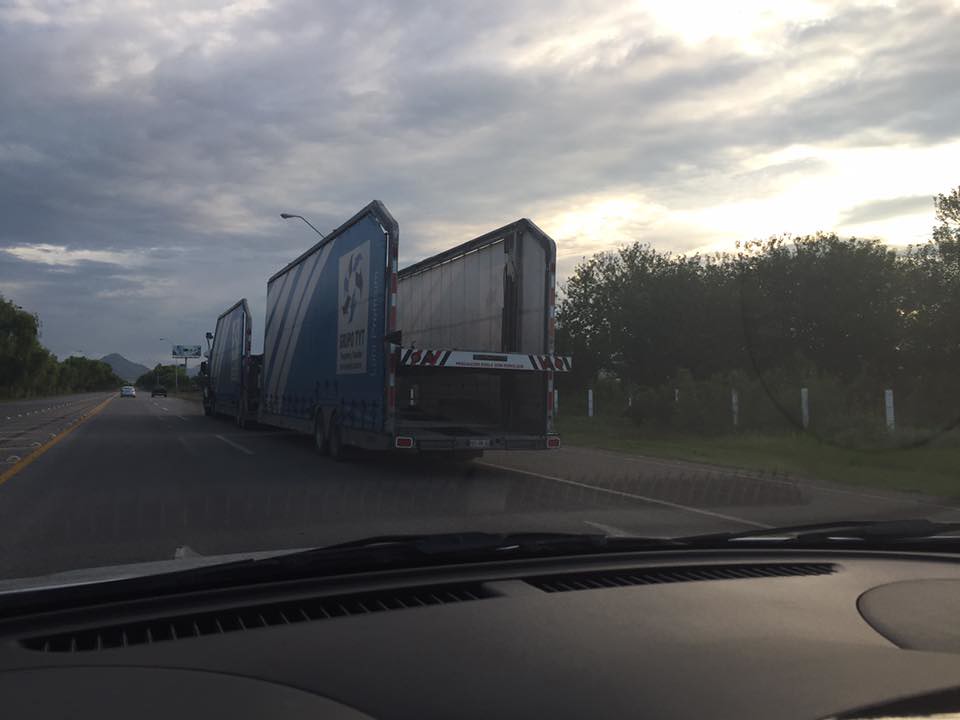This photograph, taken from inside a car, captures a scene on a two-lane highway marked by central yellow stripes and bordered by white-stripe-lined lanes. The photo prominently features a distinctive tandem tractor-trailer truck positioned slightly to the right. The truck is hauling two open trailers, each characterized by blue sides with white diagonal stripes and a conspicuous white rectangular emblem displaying a radiant pattern of arrows. The trailers, which lack a roof and back, resemble large U-shaped structures with visible straps holding the sides in place, creating an impression of flatbed trailers without any apparent cargo. The scene includes a black car ahead in the right lane and a white car further left. The highway is flanked by green grass, deciduous trees, and white bollards. Above, the sky is predominantly overcast with heavy blue-gray clouds, but a break in the clouds reveals the sun, casting a muted light over the landscape. The dashboard, windshield wipers, and a bit of the car's hood are visible at the bottom of the image, exemplifying the photo's in-car perspective. In the distance, the outline of a serene mountain range can be discerned.